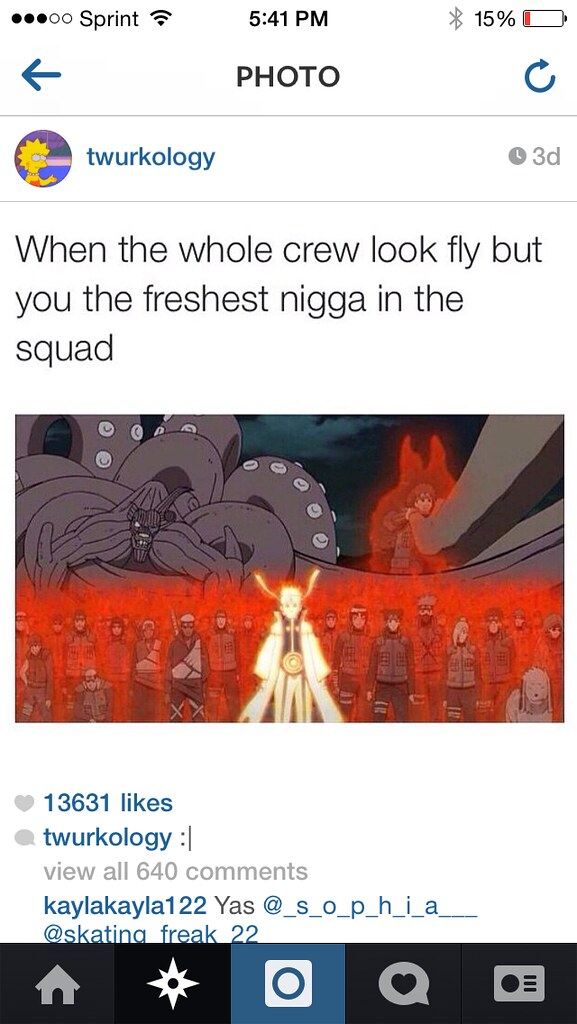In this animated image from a social media app, shared by a user with the profile picture of Lisa Simpson and the username Twerkology, there is a scene reminiscent of an anime show. The prominent figure, donning a shiny gold samurai outfit and a large medallion, stands confidently in the center. Surrounding this central character are approximately 20 warriors brandishing swords, a mix of both men and women, all depicted as slightly smaller in stature. Looming behind them is a monstrous creature with an octopus-like lower half and a menacing face, providing a dramatic backdrop. The vivid image itself retains a dark brown hue, creating a striking contrast against the more colorful elements.

The Instagram-like interface reveals that the post was made three days ago and has garnered significant interaction with 13,631 likes and 640 comments. The caption accompanying the image reads, "When the whole crew look fly, but you the freshest nigga in the squad." Instragram's familiar icons for home, photo, likes, notifications, and more are neatly arrayed at the bottom, reflecting typical social media navigation options. The top of the screenshot indicates standard smartphone details such as the Sprint network, time at 5:41 p.m., and a near-depleted battery at 15%.